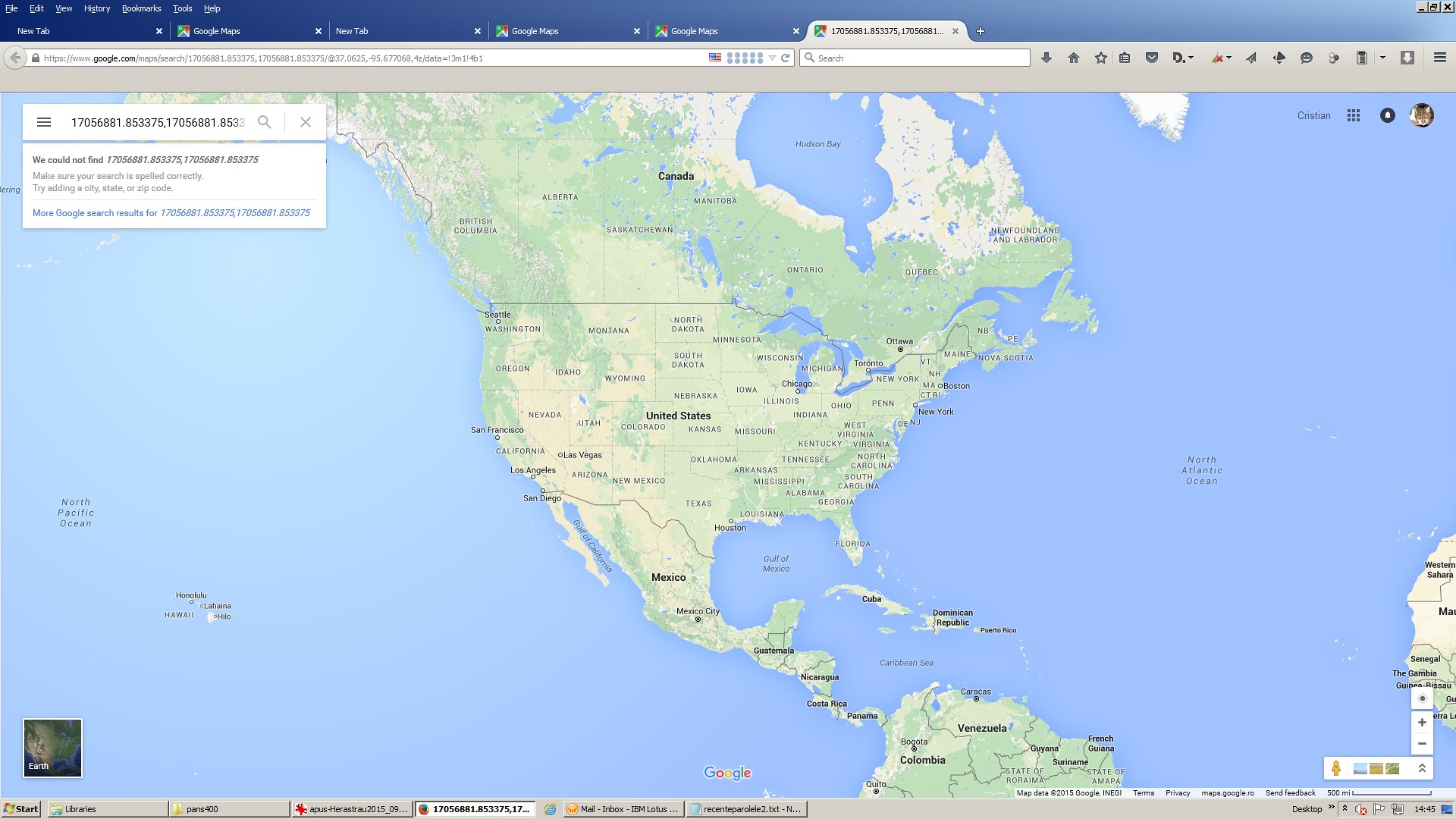The image showcases a detailed map displayed on a computer screen, highlighting geographic regions with remarkable clarity. The map prominently features the United States and Canada, with their borders and major landmarks clearly delineated. Central America is also visible, leading down to the northern part of South America, where countries like Venezuela and Colombia are identifiable despite the text being somewhat difficult to read. Surrounding the landmasses, the vast expanses of the North Atlantic Ocean and the Pacific Ocean are also captured. Additionally, there is a notable inset positioned at the bottom left corner of the screen. This inset, labeled "EARTH" in white letters, appears to be a satellite image or digital globe, consistent with a Google Earth representation, providing a global perspective within the detailed map view.